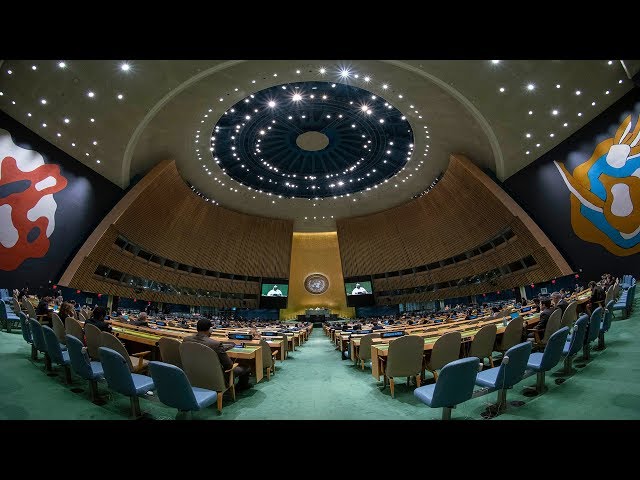The image depicts a wide-angle view of an indoor auditorium or lecture hall with staggered seating, reminiscent of a law school classroom. The ceiling features a light gray, circular design surrounded by a prominent dark blue ring, adorned with sparkling recessed lights. A lighter beige half-circle complements the circular arrangement. In the center of the layout is an aisle with green carpet leading to a centrally placed podium. The podium is set against a distinguished gold banner wall that bears a circular emblem. This emblem is flanked by two large TV screens. The room's semi-circular walls are made of distorted wood, with windows sporadically placed within the structure. On the left side of the auditorium, there’s an abstract painting with red and white blotches, whereas the right side showcases a painting with blue, yellow, white, and light brown hues. The rows of tables and chairs rise as they stretch toward the back, and at least half of the seats are visibly occupied.